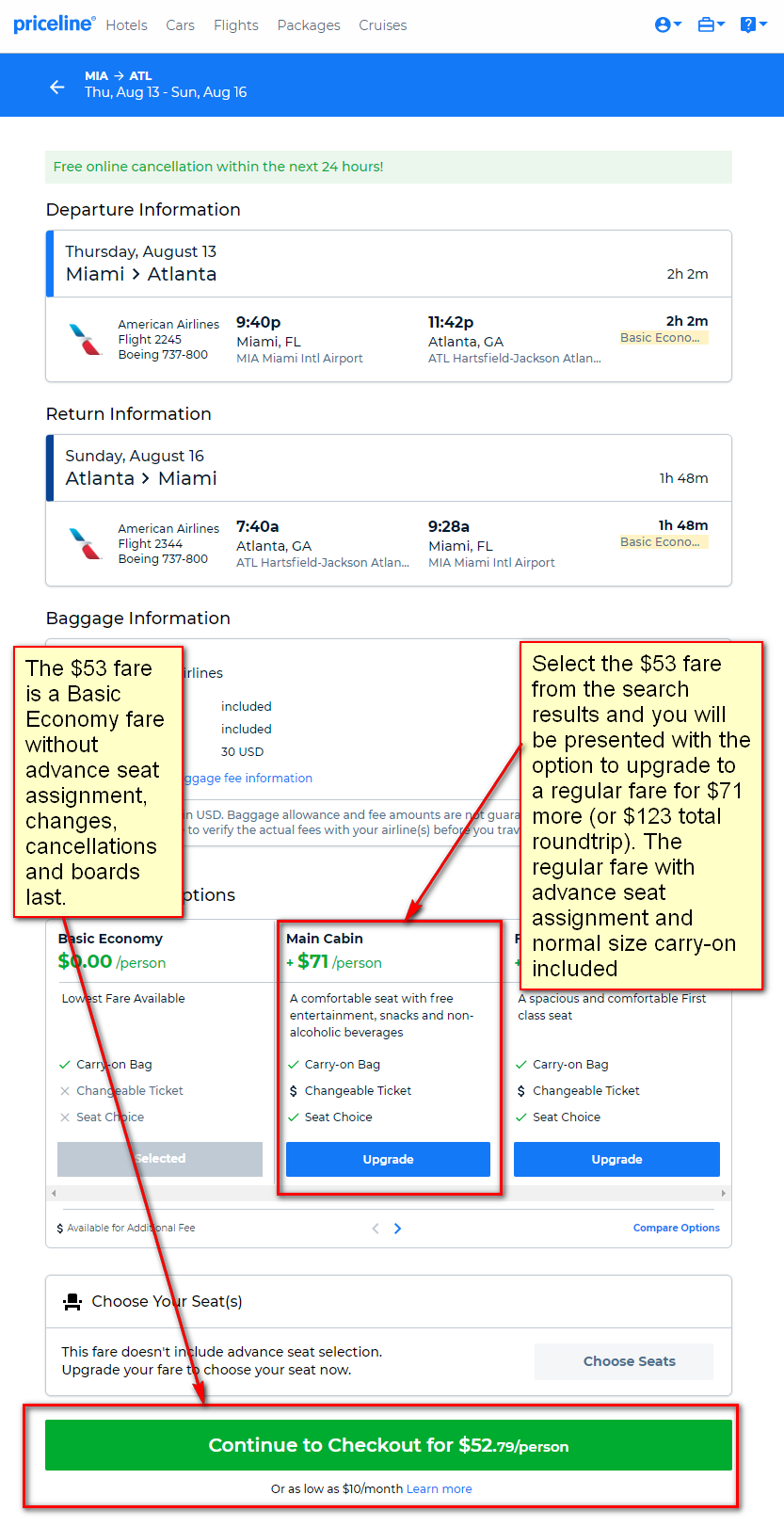Here is a detailed and cleaned-up caption for the described image:

---

The image is a screenshot from Priceline.com showcasing the departure and return details of a flight booking. At the bottom of the page, two sections are prominently outlined in red. The first section, labeled "Main Cabin," has a red arrow pointing to it with a caption that reads: "Select the $53 fare from the search results, and you will be presented with the option to upgrade to a regular fare for $71 or more, resulting in a total round trip cost of $123. This regular fare includes advanced seat assignment and a normal-sized carry-on."

The second red-outlined section is located at the very bottom and is a "Continue to Checkout" button, labeled with the fare price of $52 per person. This section also features a red arrow and a caption explaining the fare: "The $53 fare is a basic economy fare without advanced seat arrangement changes, cancellations, and boards last."

The entire page has a white background, emphasizing the flight details and the red-highlighted sections for easier navigation.